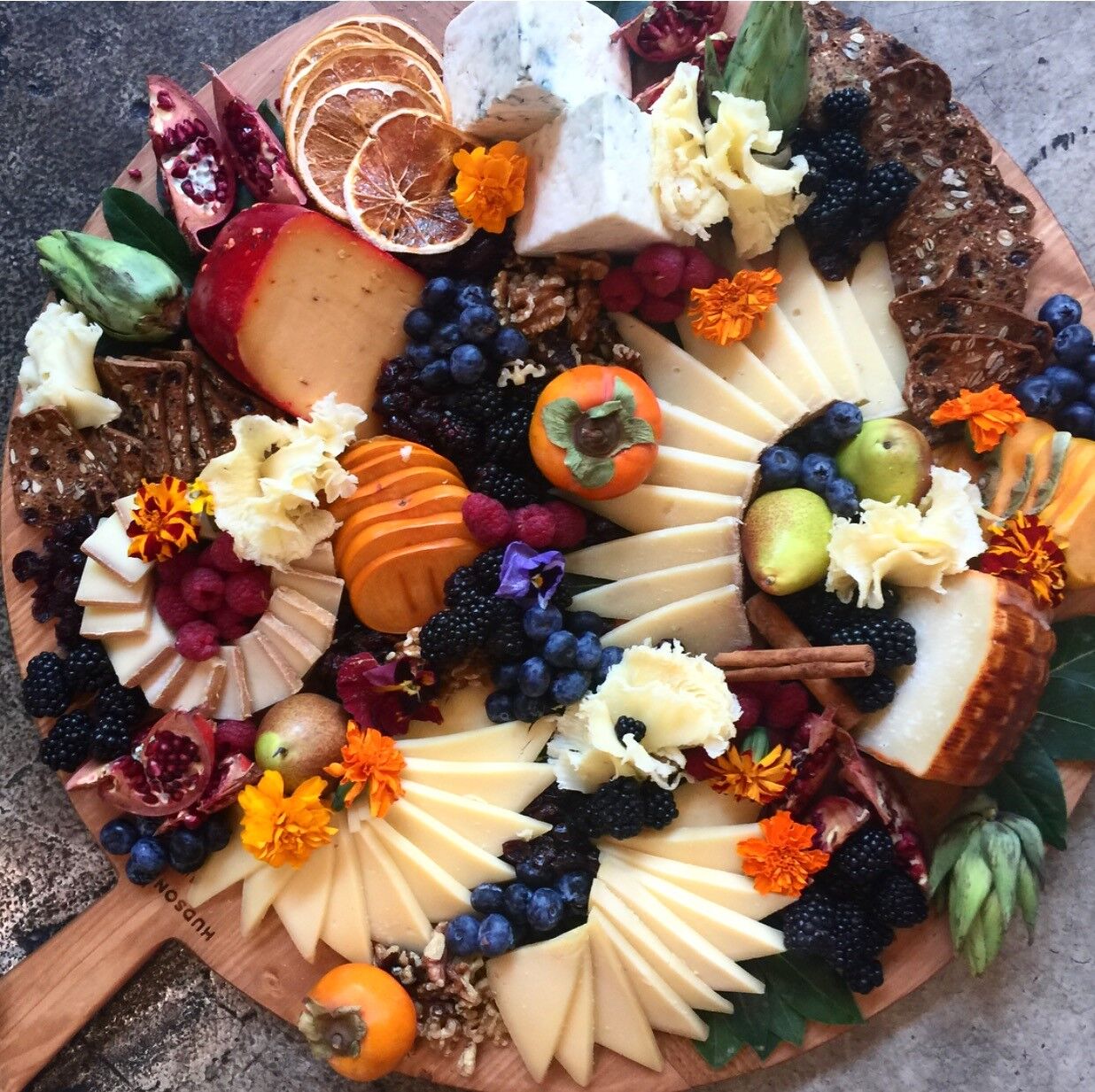This visually stunning image captures an elaborate cheese and charcuterie board displayed on a wide vertical, paddle-shaped wooden board with a round surface and a handle. The board is densely populated with a delightful assortment of foods presented in a semicircular arrangement. Various types of cheeses dominate: light yellow cheeses, wedges dipped in red wax, blue cheese, and shaved cheeses. Complementing these are soft cheese spreads. The board features an array of fruits like persimmons, blueberries, blackberries, raspberries, pomegranate seeds, sliced oranges, and tiny orange-ish yellow tomatoes. Edible flowers such as marigolds and pansies, green leaves, cinnamon sticks, and clusters of walnuts add to its vibrant appeal. Additionally, there are whole grain crackers or bread slices, artichokes, pears, and dried fruits like orange or lemon slices. This exquisite spread is set against a backdrop of a dark grey marbled stone countertop.